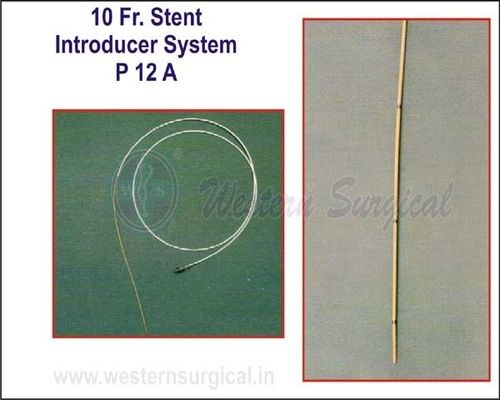The image is divided into two main sections, each showcasing medical apparatus on a white background bordered narrowly by black. In the top left, blue text reads "10 FR. Stent Introducer System P12A." Below this, a square with a red border and a green background displays a coiled thin wire, featuring a yellow end and a small metal connector. To the right, a taller rectangular box bordered in red and filled with a gray, fabric-like texture presents a long, beige tube with metal bands at three different intervals. The bottom left corner displays a light blue watermark that reads "www.westernsurgical.in," with the term "Western Surgical" stamped across the image, giving it a formal, educational presentation style. The colors in the image include a mix of purple, black and white, green, red, white, yellow, tan, and gray. The objects are positioned next to each other in a well-spaced manner.